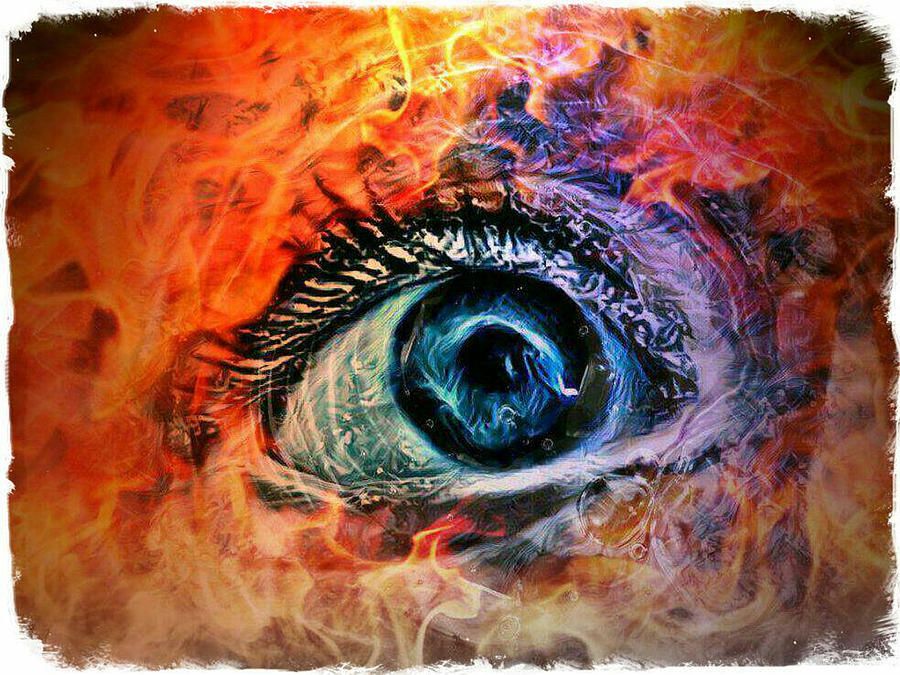This image features a striking graphic of a torn, jagged-edged rectangle, predominantly showcasing a single eye at its center. The eye, with its long black eyelashes, is wide open and appears to be looking up and to the right, evoking a sense of terror. The artistry combines elements of oil painting and digital art, giving it a textured canvas feel with semi-transparent layers adding depth. The iris is predominantly dark blue, encircled by a black ring, and contains shades of turquoise in the whites. The background is a dynamic, almost realistic depiction of flames, with vivid oranges, yellows, and reds, interspersed with smoky areas, presenting a stark contrast to the cool blues and turquoise within the eye. This juxtaposition invokes a fire and water theme, suggesting an intriguing blend of emotions and elements, further enhanced by the subtle details like bubbles within the eye, lending a surreal, stylized touch to the overall composition.